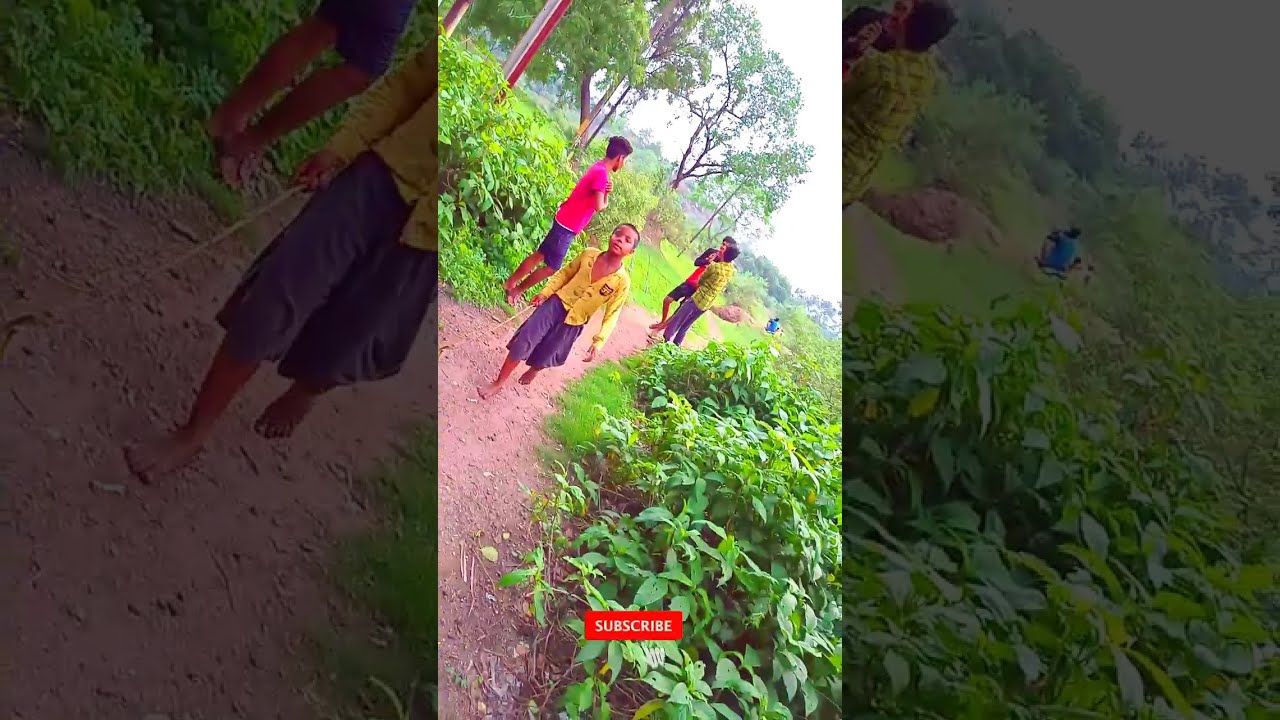This image is a wide rectangular photograph composed of a tall vertical picture in the center, flanked by close-up fragments of the same picture on its left and right sides. The central image is oriented diagonally, creating an unusual view of the scene. It captures a group of children walking barefoot down a dirt path, which is flanked by lush green plants. The foreground features a younger boy with dark skin and short hair, wearing a yellow long-sleeved shirt and blue, knee-length shorts. Just behind him to the left is a slightly taller teenage boy with short black hair, dressed in a pink t-shirt and blue jean shorts. Further down the path are two more boys, partially shown, both barefoot — one wearing a yellow shirt and the other a pink one, both paired with blue shorts. The ground beneath them appears dry, hinting at drought conditions. The repeated details and composition suggest that it might be a screenshot from a video. Across the bottom of the main image, there's a red box with the word "subscribe," indicating a call to action, possibly from an online video platform. The serene backdrop of trees and plants frames the children, who appear to be interacting and playing naturally.